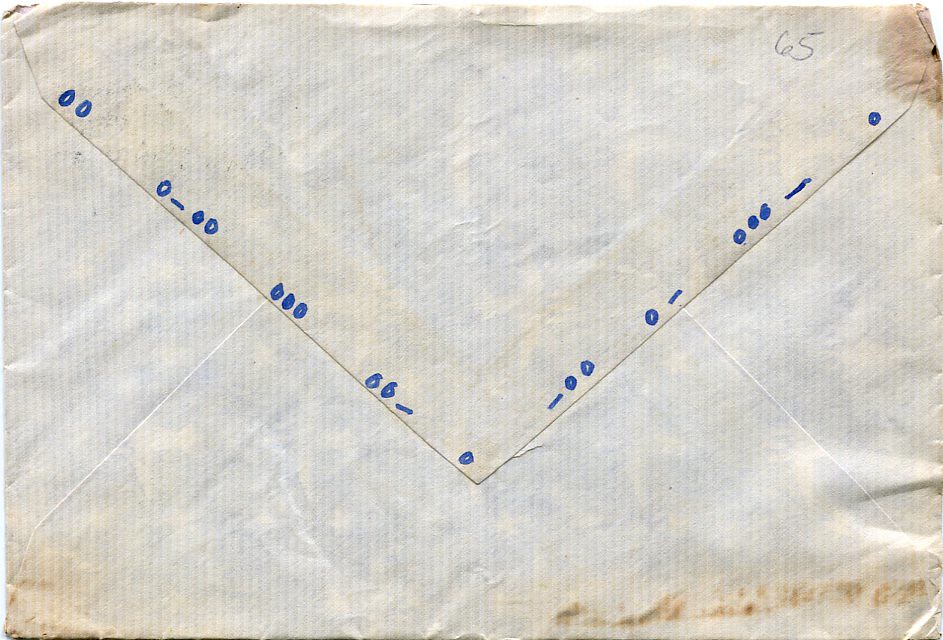The image depicts the back of a heavily worn and battered white envelope. The envelope exhibits extensive damage, with notable areas of distress including burnt or stained marks, particularly in the top right-hand corner, where a portion is missing. Various brown smears are visible along the bottom and the upper right, resembling coffee stains. The envelope appears wrinkled and bent at the corners, and its top is slightly curled. Written in blue marker, sequences of zeros can be seen on the back flap, arranged in a pattern: "00, 0-00, 000" on the left, and "minus 00, 0 minus, 000 minus 0" along the right edge, resembling some form of coded sequence. Additionally, the top right corner is marked with the number "65" in pencil, adding to the envelope's aged and distressed appearance. The markings and overall condition suggest it might once have accompanied a card, rather than being a business envelope, evoking a sense of nostalgia as it seems to have endured significant handling and possibly been kept for sentimental reasons.